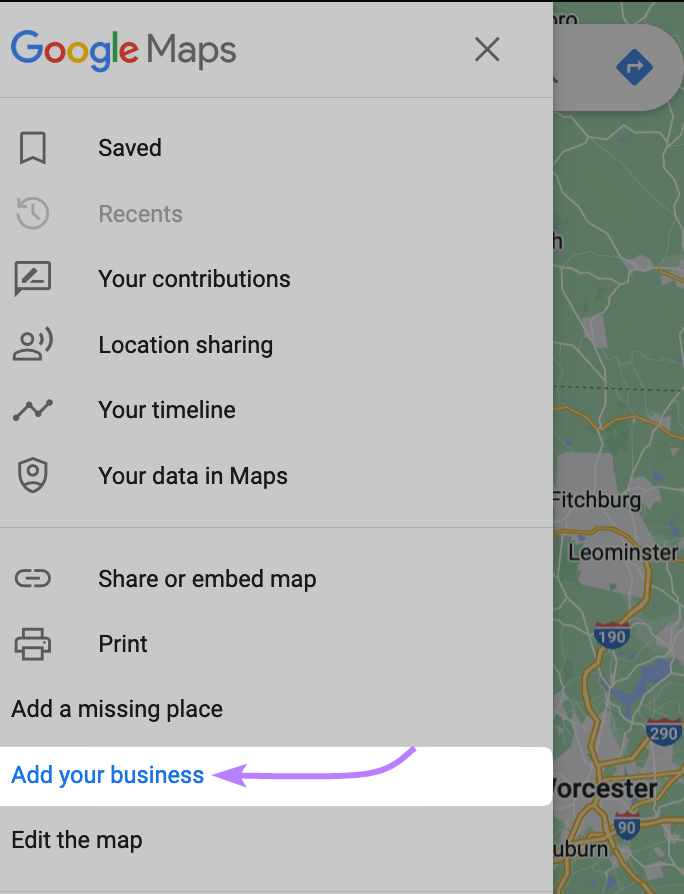The image is a screenshot of a partial Google Maps interface on a desktop or laptop computer. The display is in a portrait vertical style, suggesting it has been cropped from a larger screenshot. At the top of the interface, the familiar "Google Maps" logo is present alongside a close button. The left sidebar is expanded, showcasing numerous options including "Saved," "Recents," "Your Contributions," "Location Sharing," "Your Timeline," "Your Data in Maps," "Share or Embed Map," "Print," "Add a Missing Place," "Add Your Business," and "Edit the Map." Highlighted in blue is the "Add Your Business" option, which is further emphasized by a purple arrow pointing to it. This indicates that the screenshot is likely part of instructional materials guiding users on how to add their business to Google Maps. In the map view in the background, locations such as Worcester, Leominster, and Fitchburg are visible, suggesting the map focuses on a region in the United Kingdom, though this is not definitive.